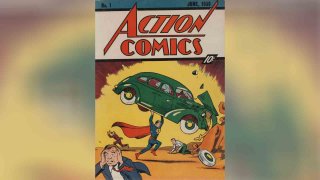This image is a detailed close-up of a vintage comic book cover from the 1950s or 60s, titled "Action Comics" in bold red letters, priced at 10 cents. At the center of the illustration, the iconic superhero Superman, clad in his classic blue suit, red cape, and red boots, is dramatically holding up a green Volkswagen Beetle-like car. His action is preventing the car from crashing into the ground. Surrounding Superman and the car are bright yellow flashes suggesting an explosion, with loose tires and pieces of the car flying off. In the foreground, people are depicted in various states of panic: a businessman clutching his face while running away and another individual on their hands and knees in fear. The chaotic scene captures the essence of action and heroism that defines classic comic book art.